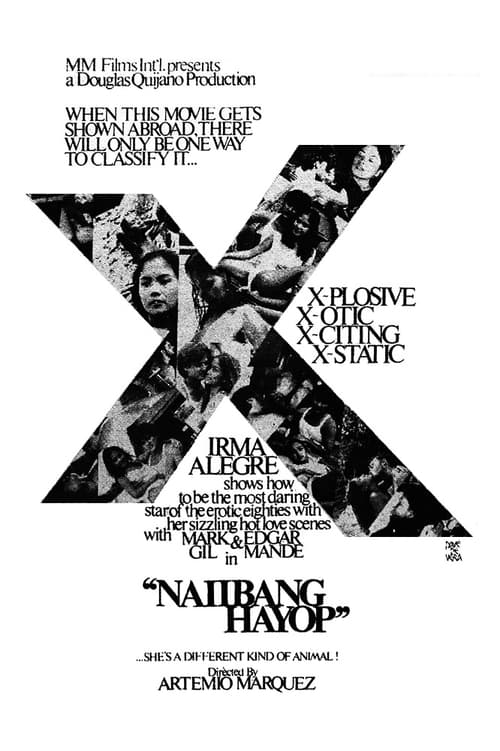This black-and-white vertical movie poster prominently features a large, slightly slanted letter "X" at its center, which is superimposed on a crowd scene with various people exhibiting different expressions and postures. Inside the "X," notable faces, including women, are visible, adding to the intrigue. Above the "X," the text reads "M.M. Films Inc. presents a Douglas DiGiorno production," setting the stage for the movie's formal introduction. 

Emphasizing its adult content, the right side of the "X" features bold words: "EXPLOSIVE," "EXOTIC," "EXCITING," and "ECSTATIC." In the middle of the "X," it highlights Irma Allegra’s role as one of the most daring stars of the erotic 80s, especially for her provocative scenes with co-stars Mark Gill and Edgar Munday in "Nayibang Hayap." The poster closes with a dramatic tagline at the bottom, "NAYIBANG HAYAP," in large black letters, drawing attention to this presumably X-rated feature, directed by Artibo Marquez.